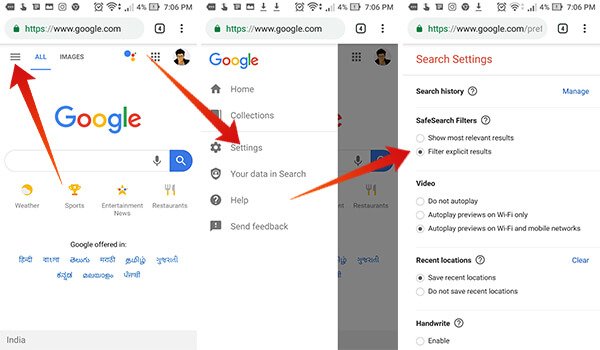The image features a screenshot of a Google desktop interface with various elements. At the top, there is a white rectangle serving as the background. Below this, there are three columns, each containing different sections.

**First Column:**
- At the top left corner, the URL "www.google.com" is displayed next to Google's icon. 
- A red arrow points upward towards three black horizontal lines that cross over the Google search icon.
- Below this, a list of categories is present: "Weather," "Sports," "Entertainment," "News," and "Restaurants."
- Further down, there is a statement "Google offered in:" followed by a selection of languages written in blue text, arranged in two rows—six languages on the top row and three languages on the bottom row.
- At the bottom of this column, a gray rectangle contains the word "India" in black letters.

**Second Column:**
- The URL "www.google.com" appears again next to the Google icon.
- A red arrow points to the word "Settings."
- Below the arrow is a menu listing: "Google," "Home," "Collections," "Settings," "Your data in Search," "Help," and "Send feedback." Each item is preceded by a black icon corresponding to its function.

**Third Column:**
- Displays "www.google.com" at the top, similar to the other columns.
- The word "Search settings" is highlighted in red.
- The rest of the text is in black, except where specified: "Search history" is followed by the word "Manage" in blue text. 
- The subsequent items are "SafeSearch Filters," "Video," "Recent Locations," "Handwrite," and "Out." Next to "Recent Locations" is the word "Clear" in blue, providing an option to clear recent locations.
- All other text items in this column are displayed in black.

Overall, the image captures a detailed Google interface with various settings and menu options illustrated with distinct colors and icons for easy navigation.